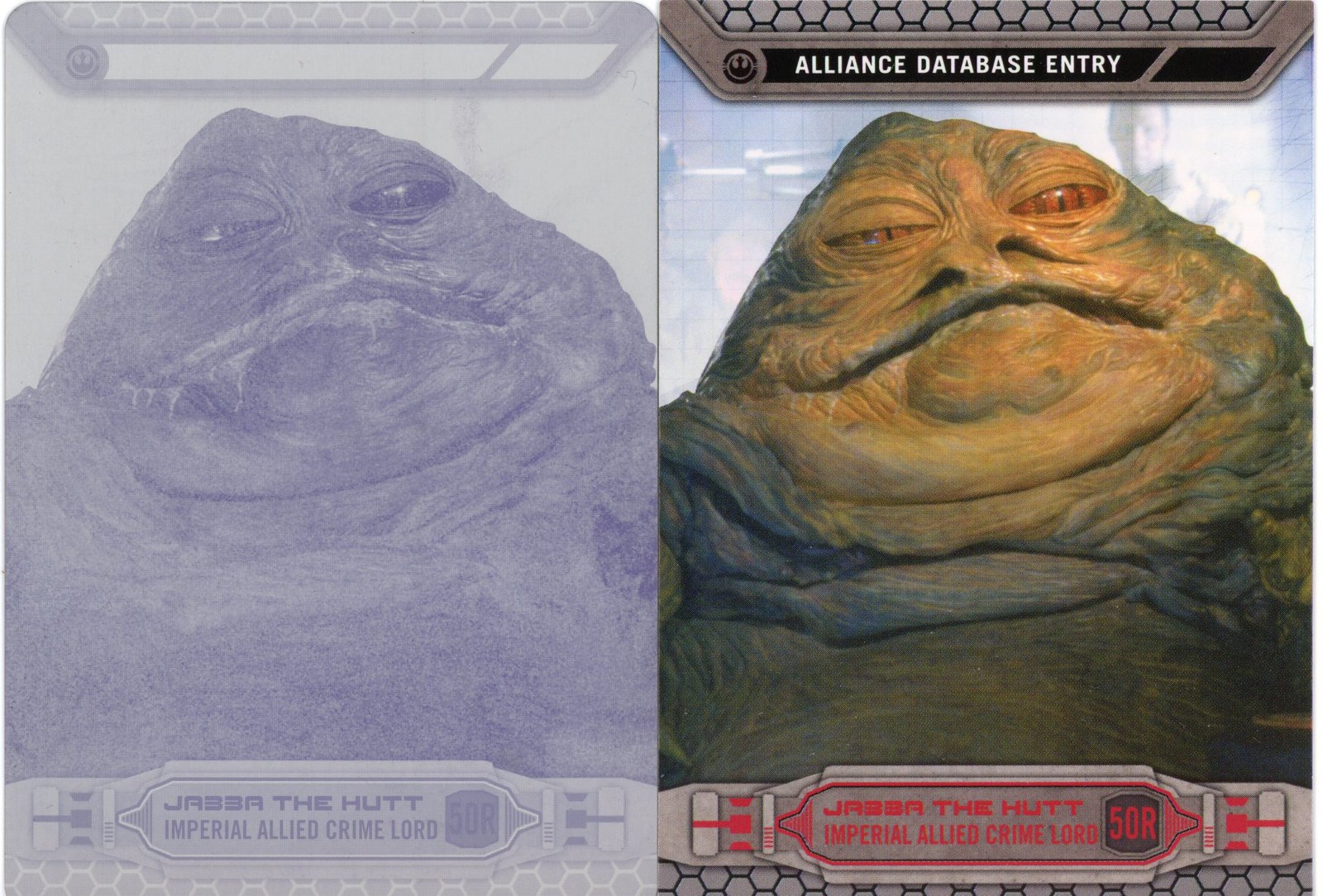The image comprises a dual depiction of the infamous Star Wars character Jabba the Hutt, resembling the interface of a video game or possibly a trading card. On the right side, a full-color close-up of Jabba reveals his greenish-yellow skin, orange-brown eyes, and partially open mouth against a hazy background, under the heading "Alliance Database Entry." Below, a red band prominently displays the text, "Jabba the Hutt, Imperial Allied Crime Lord, 50-R." On the left side, an identical image of Jabba is rendered in gray-scale, mimicking a security scan and making it challenging to discern details. Both sides contain the same text, highlighting Jabba's notorious status within the fictional universe.